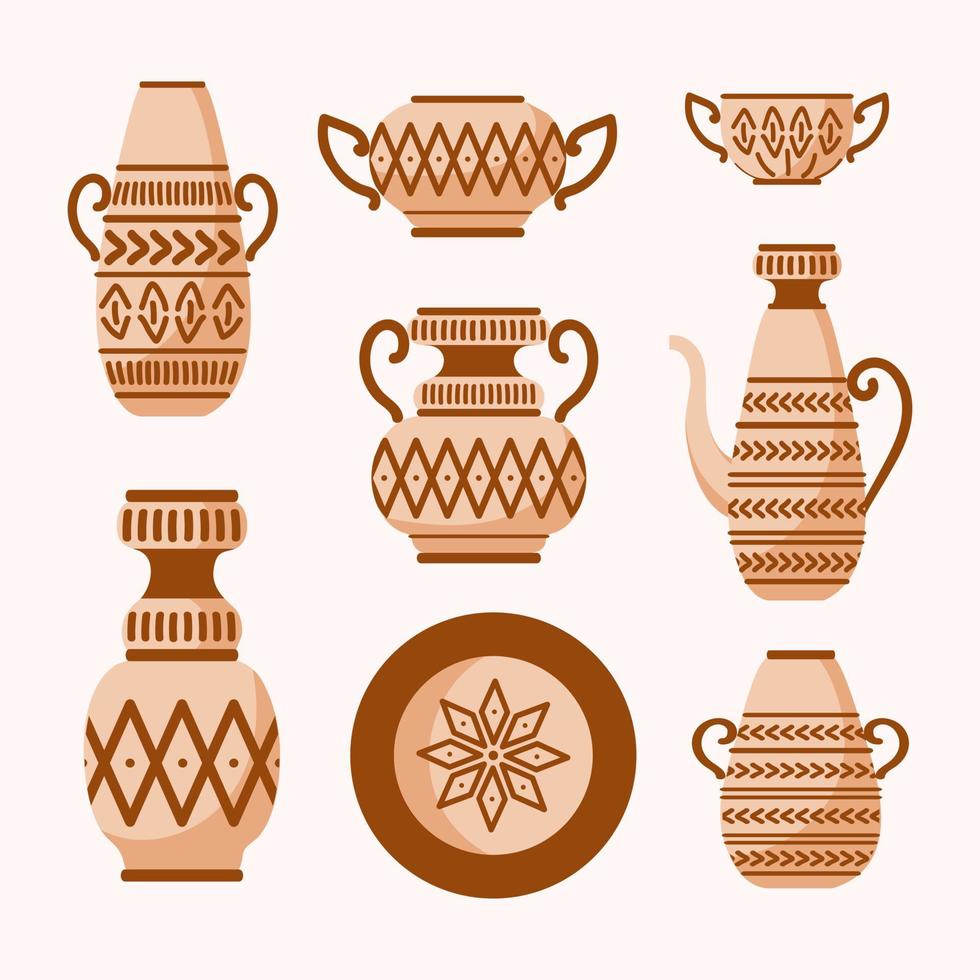This image showcases a collection of eight simplistic, illustrated pottery items including jugs, a teapot, teacups, urns, and a plate. Each object is rendered in a cohesive color scheme of light tan with brown accents. The items are arrayed on a blank white background and characterized by their two-dimensional, clipart style without shadows. Central to the composition is a plate with a star-shaped pattern and a brown border. The remaining objects, viewed from the side, display a variety of shapes and heights—some resembling teapots with spouts, while others are more urn- or teacup-like. Ornate handles, curving where they attach, and an assortment of geometric patterns, including chevrons, diamonds, and horizontal lines, embellish the pottery, contributing to their unique yet harmonious appearance.